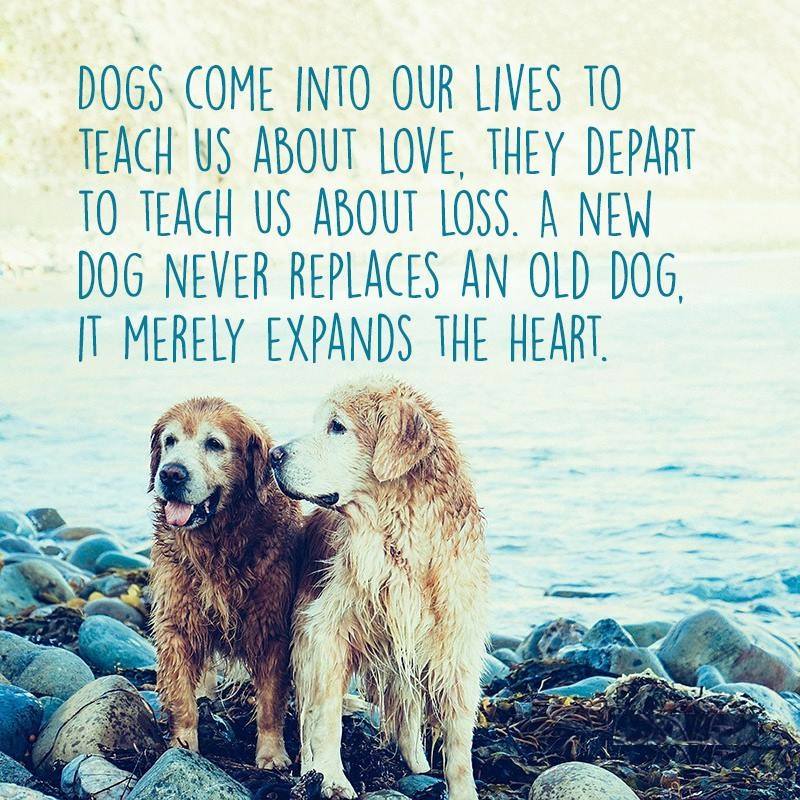In this detailed and evocative outdoor scene, two wet golden retrievers stand joyfully on a rocky shore near a large body of water, likely a beach. Their fur is damp, suggesting recent play or rain, and their expressive faces exude happiness; one dog looks off into the distance with its mouth open and tongue hanging out, while the other gazes curiously to the right. Above them, inspiring text reads: "Dogs come into our lives to teach us about love, they depart to teach us about loss. A new dog never replaces an old dog; it merely expands the heart." In the background, a majestic mountain rises near the water, enhancing the natural beauty of the scene. The bright colors and daylight indicate it's taken outdoors in the middle of the day, making this image a perfect motivational meme to share online.